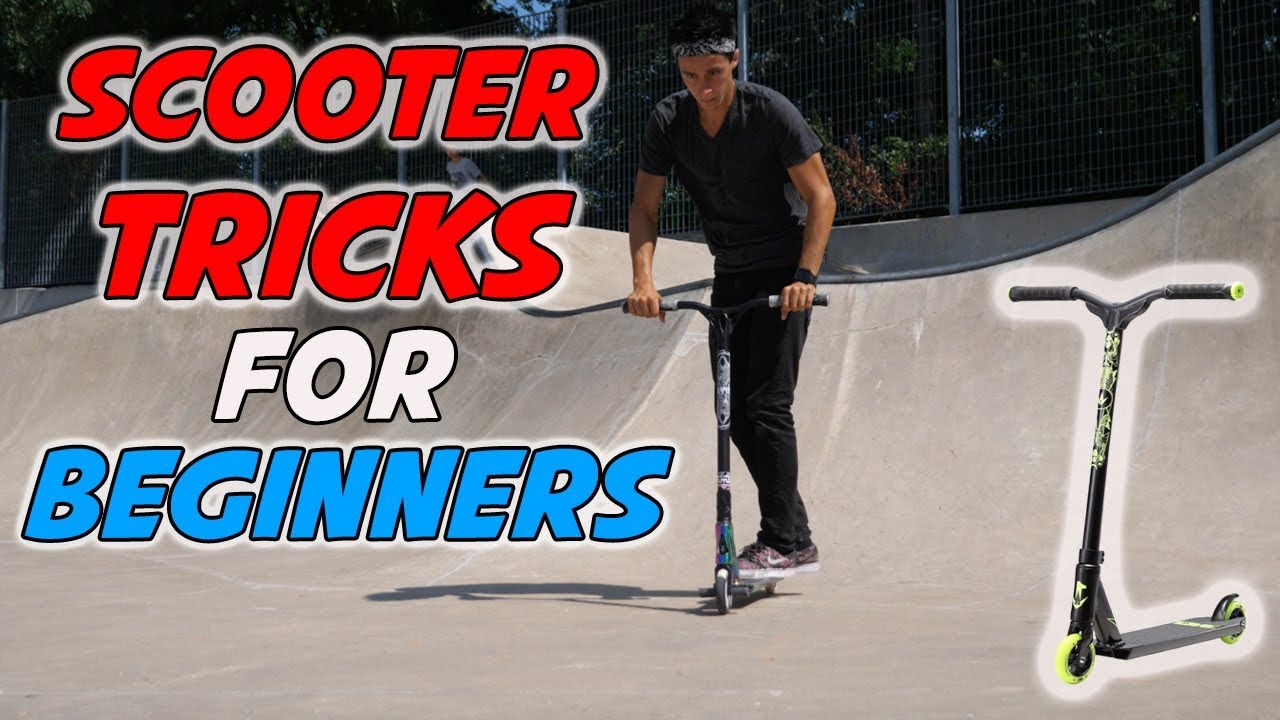The image captioned "Scooter Tricks for Beginners" features a young man riding a manual scooter down a slope at a skate park. The scooter he is riding is black with white details and green accents just above the wheels. He is dressed in black pants, a black short-sleeved t-shirt, and sneakers, and is focused on his descent, with both hands gripping the handlebars. To the left side of the image, italicized text reads "Scooter Tricks" in bold red with a white outline effect. Beneath it, the word "for" is displayed in white with a solid black outline, and "Beginners" appears in blue with the same white outline effect as "Scooter Tricks." Additionally, on the right side of the photo, there is a superimposed image of another scooter, predominantly black with neon green details and light neon green wheels, suggesting an advertisement element. This secondary scooter mirrors the simple design of the one being ridden.